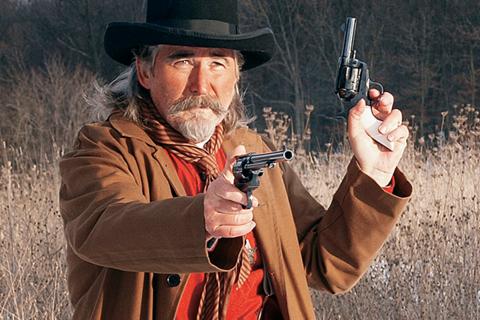The image is a photograph, potentially from a TV show or movie, taken outdoors during the daytime. It captures an older Caucasian man standing slightly left of center, framed from the waist up. His appearance is distinctly old-western, characterized by slightly longer salt-and-pepper hair, bushy gray eyebrows, and a pointed gray mustache and beard. He wears a black brimmed cowboy hat, a brown overcoat, and a red shirt underneath. Around his neck is a light tan and red striped scarf. The man holds a pistol in each hand; his right arm extends forward, aiming the pistol directly at the viewer, while his left arm is bent at the elbow with the pistol pointing upwards.

The backdrop features a natural, unkempt setting that appears to reflect autumn. Tall, dead grass with seed pods dominates the lower half, transitioning into a sparse tree line with slender, mostly leafless branches in the upper half. The combination of the man’s old-western attire and the rustic, fall scenery suggests a scene evocative of historical drama or a period piece.